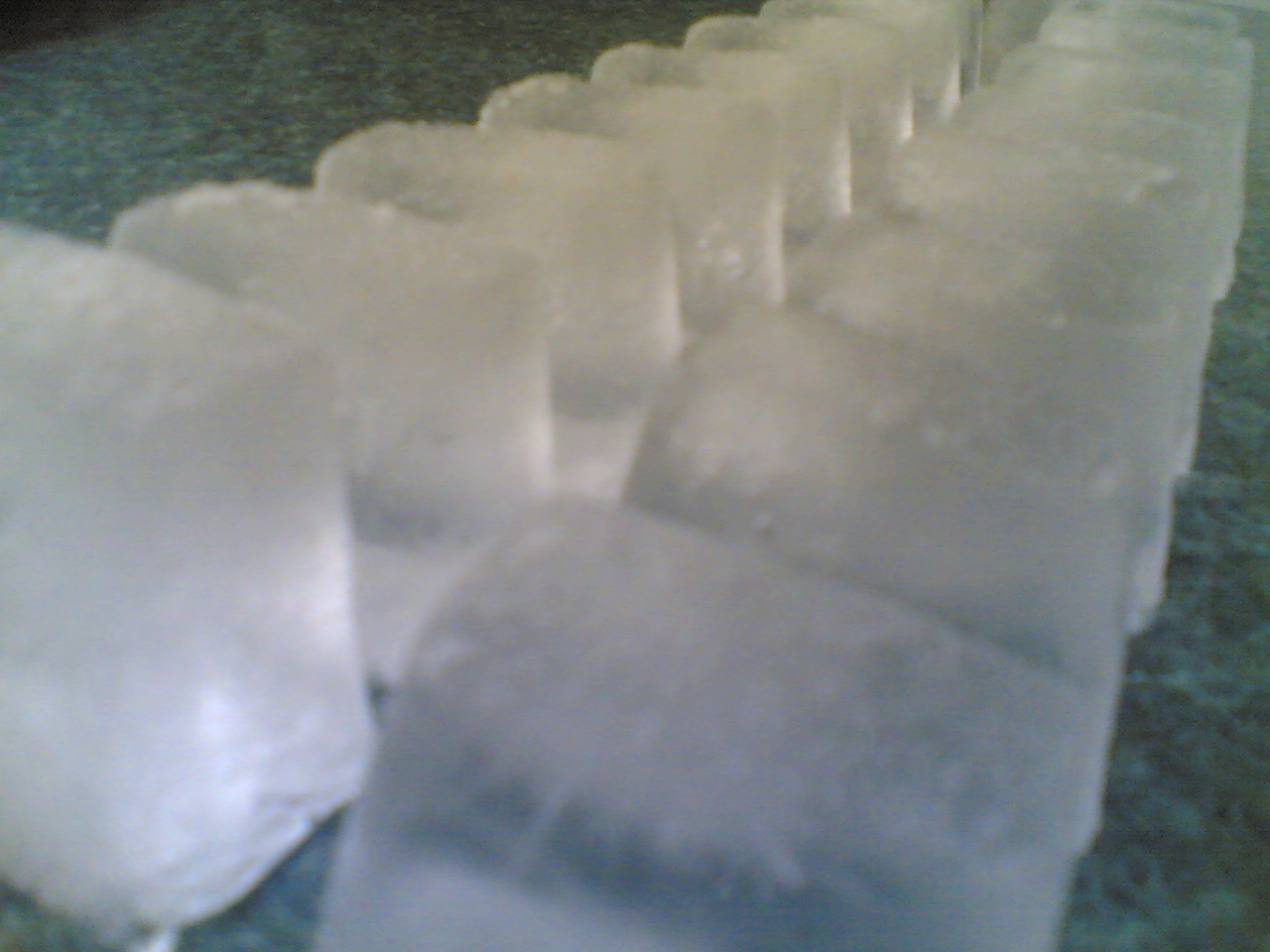This is an extreme close-up photograph featuring two neat rows of ice cubes placed diagonally from the lower left to the upper right on a green speckled countertop, which appears to be granite. The cubes, likely just released from an ice tray, are all uniform in size and neatly aligned as if the tray was flipped directly onto the counter. The image, though grainy and blurry, captures at least eight to nine cubes in each row, blending together towards the back due to the zoomed-in perspective. A subtle light source from the left highlights the cube in the lower left corner, adding a slight glow to its otherwise hazy appearance. The countertop features a green marble-like design with lighter and darker green speckles. Despite the close-up nature of the photo, there's no sign of melting, and no water is visible, indicating the ice cubes are well-preserved in their current state.